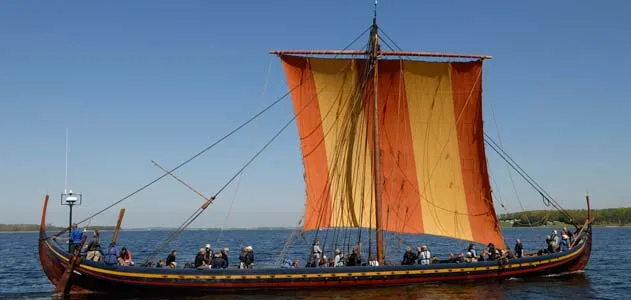This is a detailed side photograph of a long, old-style wooden sailboat that resembles a Viking longboat. The vessel, reddish in color, is elongated and canoe-like, featuring a large, square sail with vertical stripes in shades of orange and yellow. The boat is populated with around 22 to 30 people, evenly distributed along its length, some appearing to be conversing. The background showcases a clear, sunny day with the horizon visible, including land on the right-hand side, indicating the boat possibly being in a bay. The sail is fully extended, prominently displaying its vivid colors against the sky. There's also a small blue and white feature at the end of the boat, resembling an antenna.